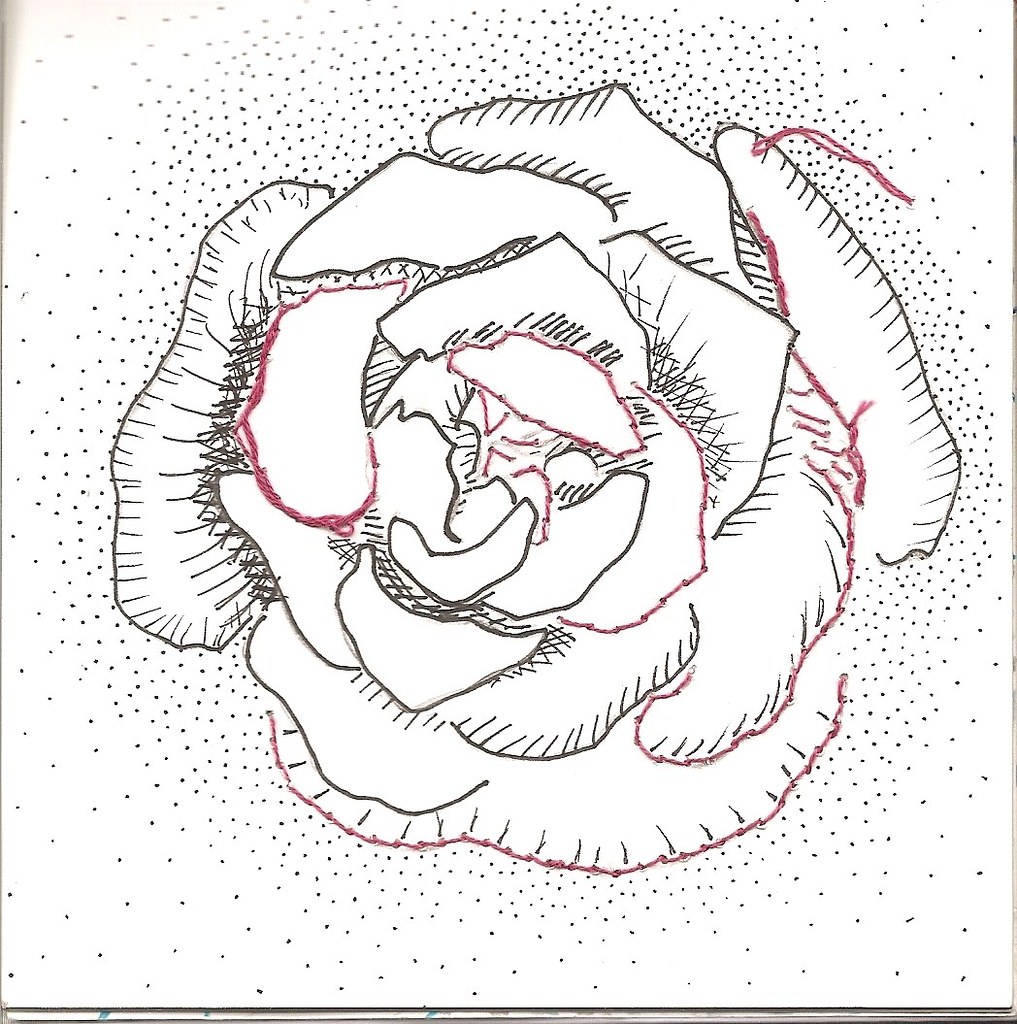This black and white drawing of a rose on white paper showcases a beautifully detailed bloom at its center. The petals are meticulously drawn, revealing intricate inner structures. Notably, there are selective accents of red that enhance the monochromatic theme: a red petal outline extends towards the right, another fully outlined petal appears on the left, and intermittent red lines accentuate areas towards the upper right and interior right petals. The artist has employed cross-hatching techniques on the lower petals to convey an unfolding effect. Surrounding the rose, a myriad of small dots, densely clustered near the flower and thinning outwards, adds depth and texture to the composition.